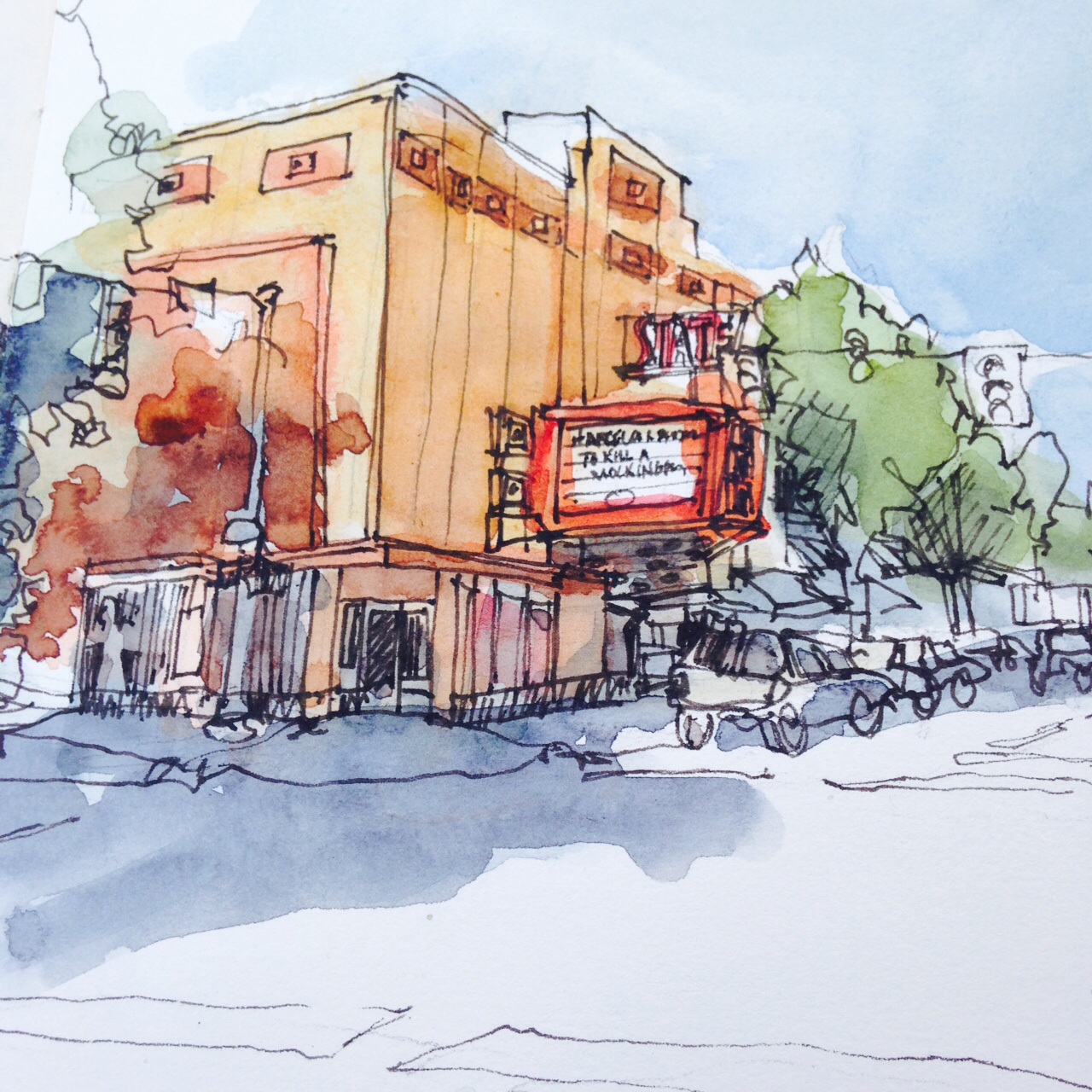The illustration is a detailed, ink and watercolor depiction of a vibrant city street. The focal point is an orange-colored corner building, which appears to be a vintage movie theater. Attached to the theater is a striking red sign with a white background, displaying the title "To Kill a Mockingbird" in black text. The street is lined with green trees that have lush leaves, contributing to the lively atmosphere. The sky, painted in hues of light blue, is slightly cloudy, indicating an outdoor setting. The street below is a light gray or blue-gray, populated with parked and moving cars which add a touch of realism despite their simple sketches. Additionally, there are detailed streetlights and a traffic light, enhancing the urban feel of the scene. The combination of cartoonish elements and meticulous details creates a captivating and nostalgic portrayal of a cityscape centered around a classic theater.